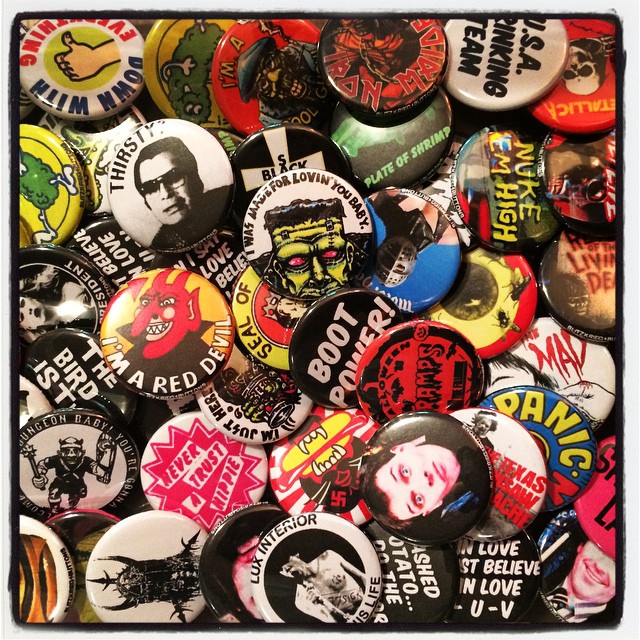The image depicts a vibrant, vertical rectangular collection of pin-on buttons piled densely upon one another, framed in black. Each button is unique, featuring a variety of bold, multicolored designs, characters, and texts. Among the most noticeable are several distinctive badges: one in the top row with the caption "Down With Everything" paired with an image of a thumb, an Iron Maiden pin, and a USA-themed button. Another prominent line showcases a yellow button depicting a green pickle with legs, alongside a pin that reads "Thirsty" featuring a character donning sunglasses against a white background. Further featured are various whimsical and eclectic buttons such as one reading "I Was Made For Loving You Baby," a badge with "Plate of Shrimp" and a question mark, and a collection labeled "Nukem High" and "Boot Power." Notably, a pin with "I'm a Red Devil" sports an image of a devil with a red head and black cape, amid a plethora of other miscellaneous designs, including slogans like "Never Trust a Hippie" and whimsical characters. The entire array suggests a rich tapestry of cultural and humorous references, capturing a snapshot of eclectic pop culture and personal expression.